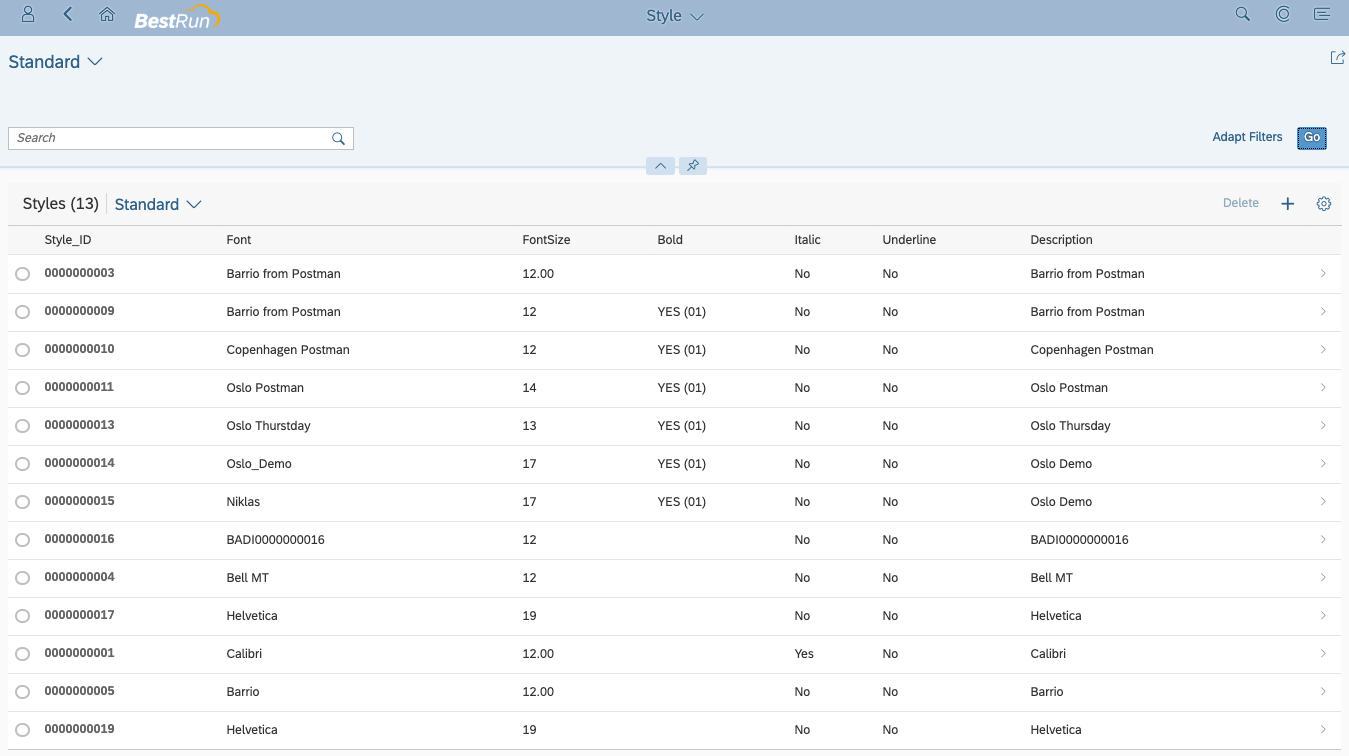The screenshot captures an interface from a website or application named "Best Run." In the top left-hand corner, there are navigational icons: a back key and a home key. Adjacent to these icons is the site's name, "Best Run." Centered at the top of the interface, there's a dropdown menu labeled "Style" with a downward arrow, allowing users to select different styles.

The main body of the interface displays an extensive list of fonts. Each font is presented in a structured format that includes a style ID, a lengthy alphanumeric code close to 10 digits. To the right of each style ID, the font names are listed. Further details about the fonts are provided to the right, including font sizes and additional descriptions indicating whether the font is bold, italic, or underlined. Some of the fonts are standard types commonly found in document editors like Microsoft Word. This detailed layout allows users to quickly compare and select fonts based on their specific attributes and styles.